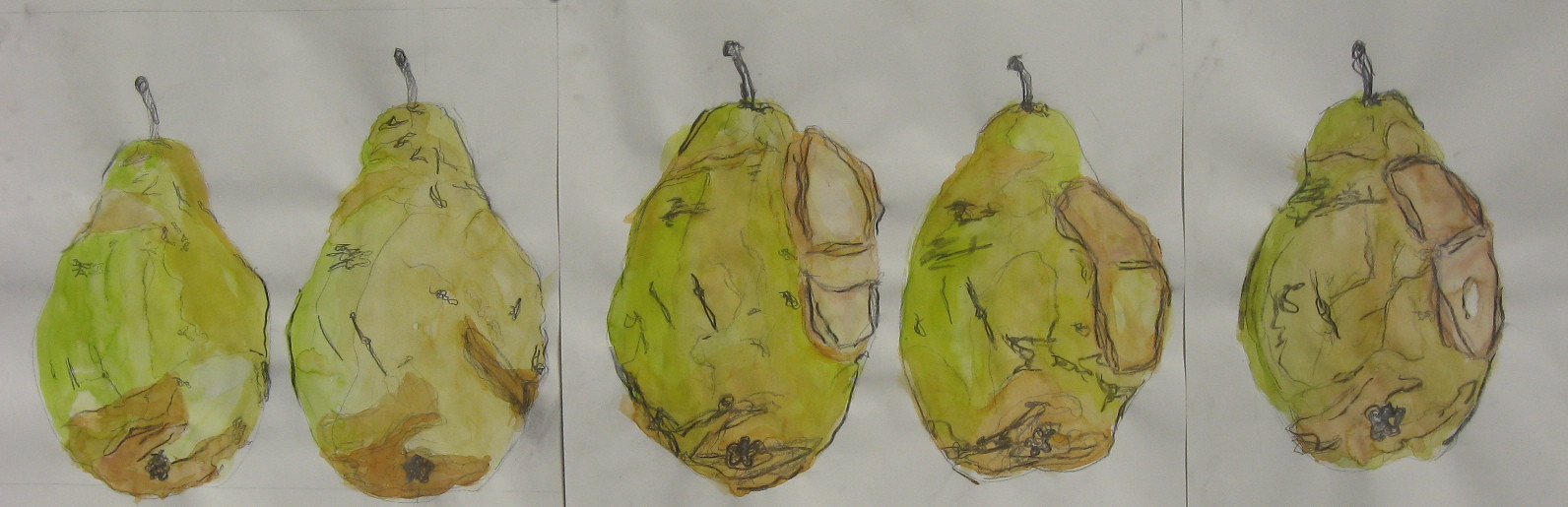This is a close-up series of five hand-drawn, expressionistic illustrations depicting the stages of a pear's ripening and decay. Each of the five images shows a pear progressing from fresh to deteriorated. 

In the first drawing, the pear is primarily green with light brown near the bottom, accented with gold and yellow highlights, and features a small white splotch. The second drawing shows the pear softening in color, with the light brown diminishing, the right side transitioning to tan, and the bottom colors becoming less harsh and more subtle. 

By the third drawing, any areas resembling damage on the pear appear to have "healed," resulting in a predominantly green pear with a small tan growth on the right side, reminiscent of a tumor in shape. The fourth image continues this transformation, with the tan growth shrinking to a finger-like shape, and tan sections becoming more pronounced at the bottom.

In the fifth and final illustration, the pear appears more shriveled, with a noticeable increase in tan areas on the body and a small white circle emerging where green once was, outlined in black. Across all drawings, the pears feature black stems, highlighting their top. The illustrations vividly capture the pear's transformation from ripeness to decay.